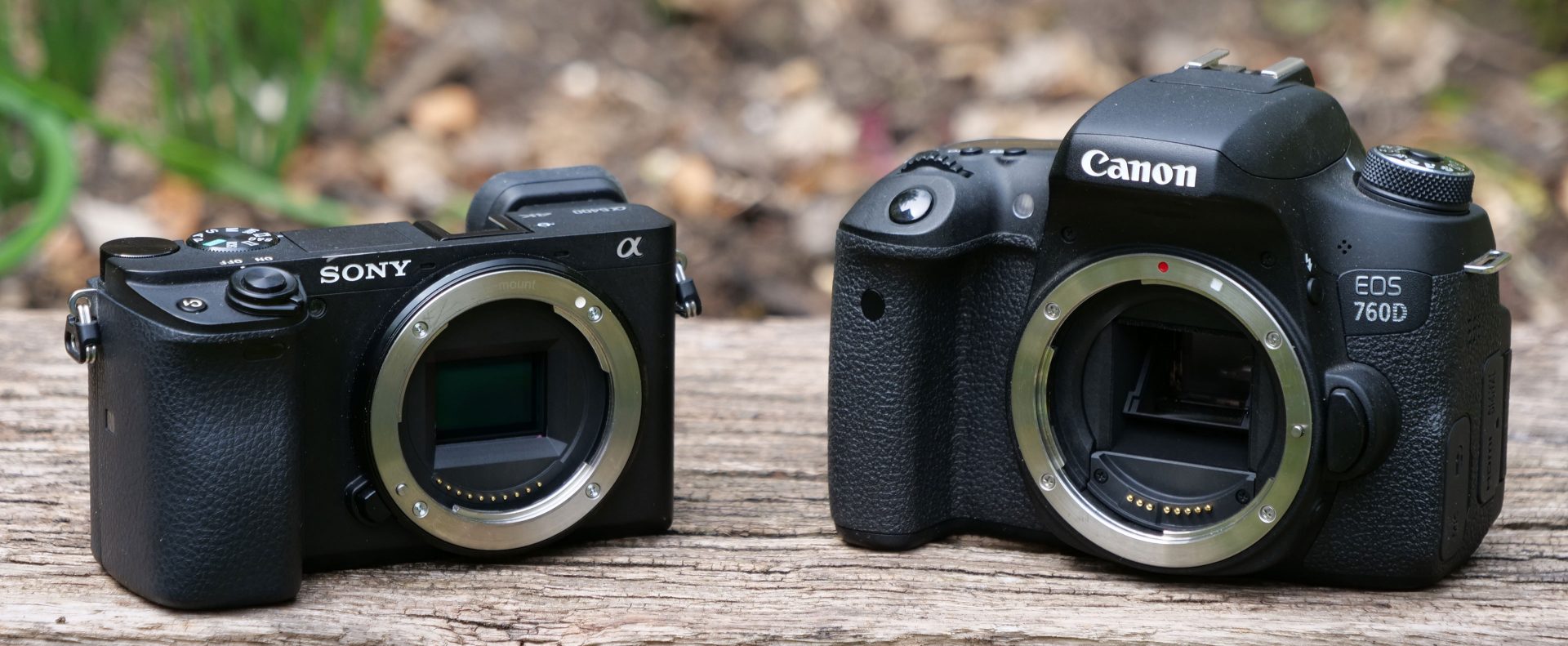In the photograph, two high-end single-lens reflex (SLR) camera bodies are prominently displayed on a dry, gray wooden log. The camera body on the left is a Sony, distinguished by its black body with a silver-framed aperture, small square lens opening, and various black buttons and attachment points for a strap, accented by gold dots above the silver part. The camera on the right is a slightly larger Canon, labeled with "Canon" across the top in white and "EOS 760D" on the right side. It too features a silver-framed, slightly tilted square aperture with gold dots above it, along with its own array of black buttons, levers, and a red dot. The two cameras are angled slightly towards each other. The background is out of focus but reveals a forest floor with brown leaves, yellow, tan, and red rocks, green grass stalks, and patches of black dirt, contributing to the natural setting of the scene.